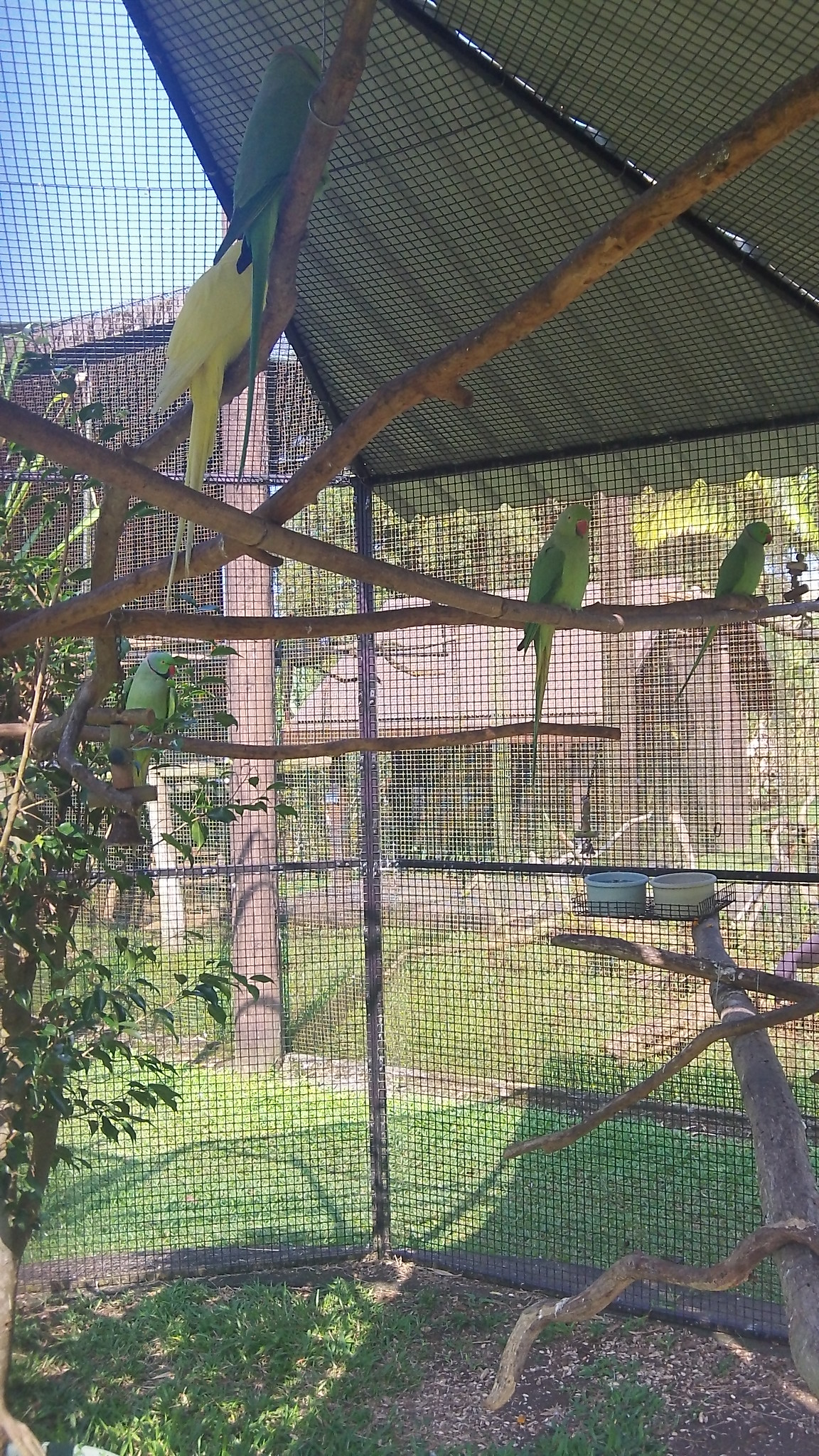The image is a vertically rectangular photograph taken from within a large, man-made avian enclosure, possibly at a zoo or conservatory. The cage features square-grid mesh sides and a partially solid roof to provide shade. Inside, five birds are perched on various wooden branches that extend across the scene. Four of the birds are predominantly light green with darker green feathers and orange beaks, while the fifth bird is a distinctive yellow, visible only from the back. The enclosure is surrounded by vegetation, with green leaves visible on the left, and grass and dirt covering the bottom. Additionally, white containers, likely for food, are scattered within the cage. In the background, architectural structures and trees can be seen outside the cage, with a glimpse of blue sky and sunlight filtering through, casting shadows within the enclosure.